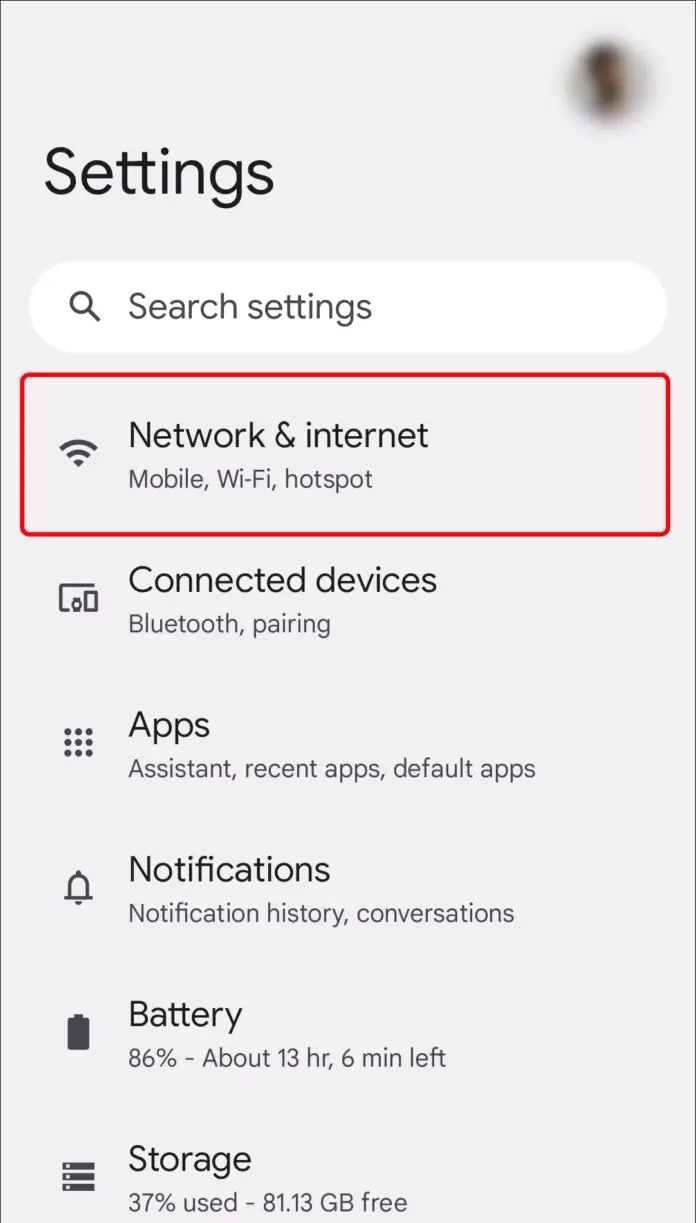The image showcases a detailed view of a settings page with a light grayish background. In the upper right corner, there is a circular area where a profile picture would typically be displayed, but the image is blurred out, making the face unrecognizable. At the top of the page, the word "Settings" is prominently displayed in black text.

Below the title, there is a white search bar featuring a black magnifying glass icon and the placeholder text "Search settings". The first section under the search bar is labeled "Network & Internet". The section includes a Wi-Fi symbol on the left and the options for "Mobile, Wi-Fi, Hotspot". This section is outlined in a red square, indicating it is currently selected.

Following this, the next section is "Connected devices" which includes options like "Bluetooth, Pairing" and shows an icon representing connected devices. Below that, the "Apps" section lists options such as "Assistant, Recent apps, Default apps" and is accompanied by an icon of nine dots arranged in three rows of three.

The "Notifications" section is next, detailing options for "Notification history, Conversations" and features a bell icon. Subsequently, the "Battery" section displays the current battery level at 86%, with an estimated 13 hours and 6 minutes of usage remaining. This section includes a completely filled black battery icon.

Lastly, the "Storage" section reveals that 37% of the storage is used, with 81.13 gigabytes still available, symbolized by a trio of horizontal lines.